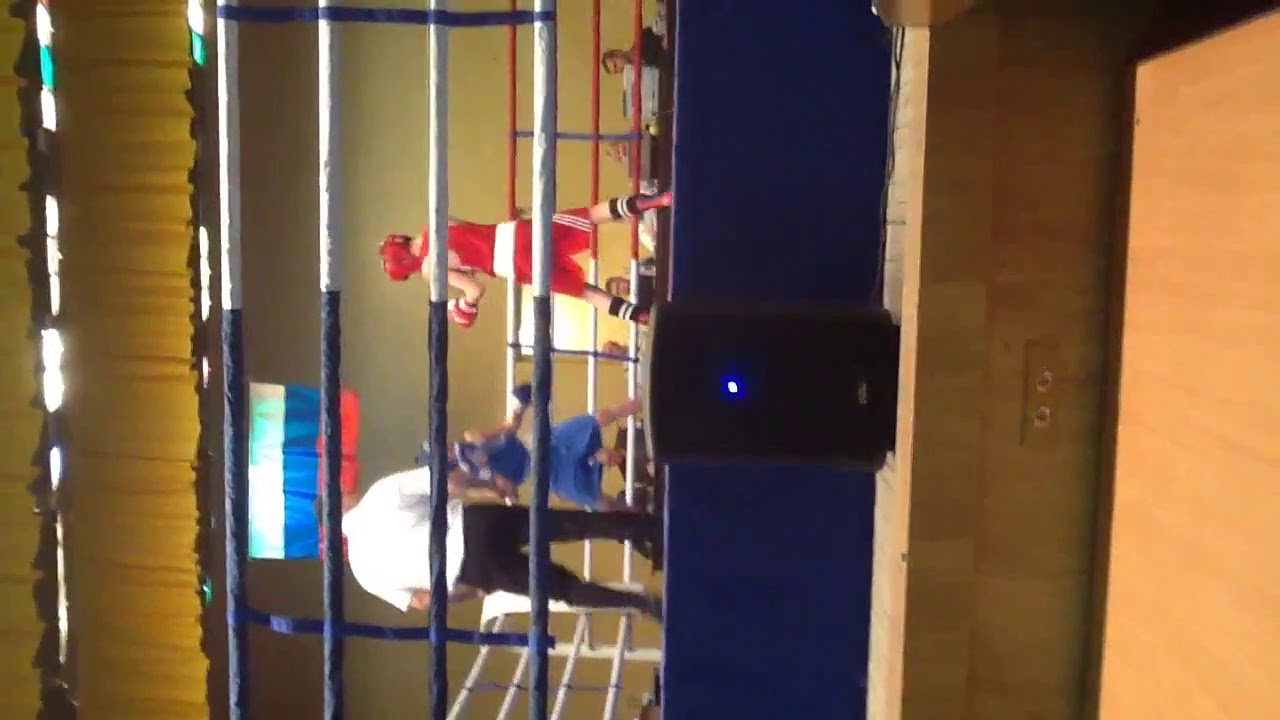This image depicts a sideways view of a boxing ring, as if the camera itself is turned 90 degrees to the left. At the bottom of the image, you see brown steps leading up to the ring, upon which sits a black rectangular speaker with a blue light glowing in the middle. As you move up from the steps, you encounter the boxing ring. The ring has four ropes—black ropes on the left side and white ropes on the right. Inside the ring, there are two young male boxers and a referee. The boxer on the right side is dressed in a complete red uniform: red headgear, red gloves, red shirt, and red shorts. His opponent, on the left, is similarly outfitted but in blue. The referee, positioned towards the back of the ring, is wearing a white shirt and black pants. The floor of the boxing ring is blue, and in the background, a flag featuring red, white, and blue colors, possibly representing a European country, hangs on the wall. Above them are gold curtains and ceiling lights, adding to the scene’s ambiance.